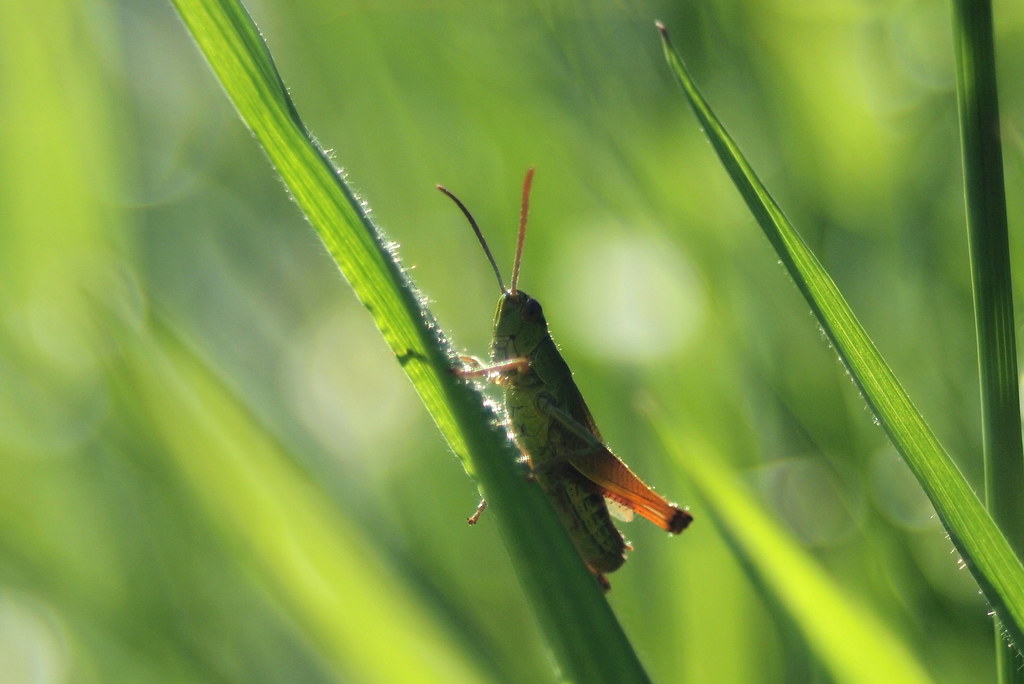The image features a close-up shot of a vivid green grasshopper, primarily positioned in the center, perched on a green leaf or stem. The grasshopper's striking details include two antennas and a noticeable orange tinge on one of its legs, a part of its wing, and an antenna. The photograph is so closely zoomed in that one can see the minute fibers on the leaves. The background consists of a beautifully blurred mixture of greens, likely representing out-of-focus blades of grass, with three distinct pieces of grass in focus. Small light dots and streaks in the background suggest sunlight filtering through, adding a natural, vibrant ambiance to the scene. It’s a nature picture with no text or other objects, emphasizing the grasshopper amidst the lush greenery.